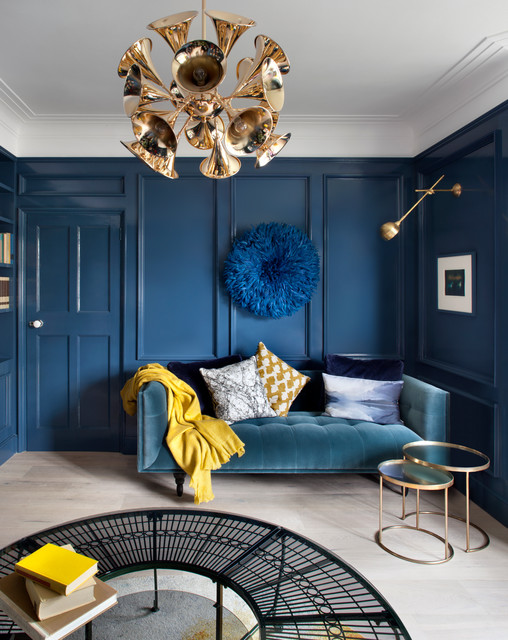The image depicts a stylishly designed room that combines modern elements with unique décor. The room features blue walls and a white ceiling adorned with elegant molded borders. Hanging from the ceiling is a distinguished chandelier that resembles golden trumpet bells. The blue wall in the background is highlighted by a blue yarn wreath. To the right of this wall is a picture and a gold lamp that extends from the wall, then bends towards it.

In front of the back wall is a luxurious blue velvet couch, equipped with a variety of throw pillows in white, blue, and brown hues, and a yellow blanket draped over its left armrest. To the left of the couch is a blue door, consistent with the room's color scheme. A pair of round tables with bronze or gold molding are situated in front of the sofa.

On the floor, featuring a light hardwood with a subtle grayish tint, there is a white rug adding a touch of coziness to the space. The lower left corner of the image captures a black semi-circle mesh table, which holds several books, including a noticeable yellow one atop the stack. Adjacent to the left wall appears to be a bookshelf, contributing to the room’s balanced and stylish aesthetic.